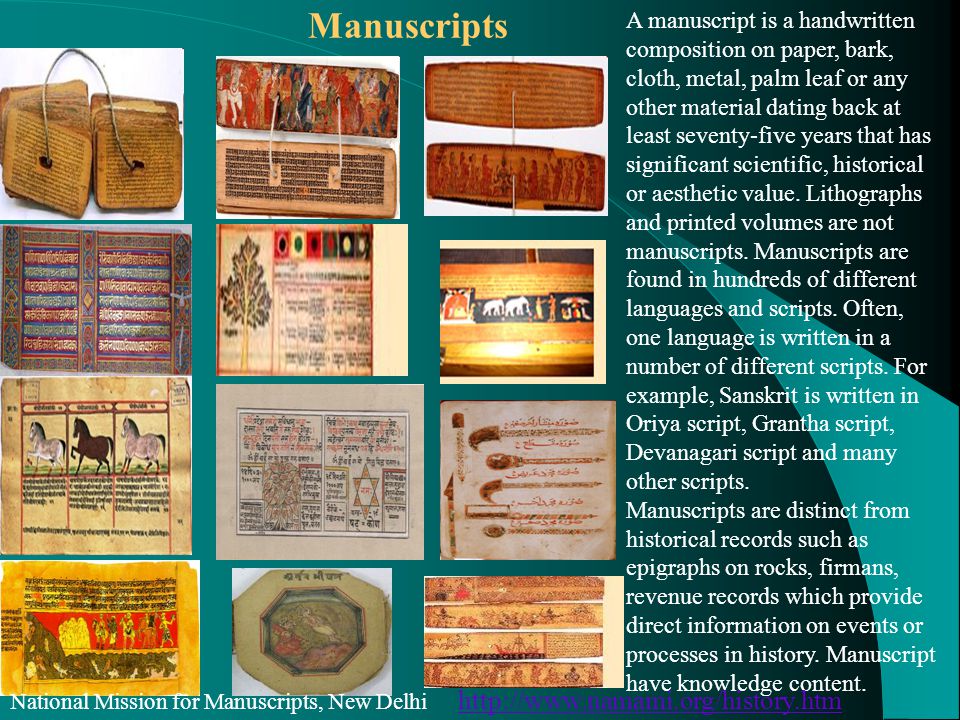The image appears to be a detailed slide or thumbnail from the National Mission for Manuscripts in New Delhi, featuring information about manuscripts. The background is green or teal with some effect underneath, and the text “Manuscripts” is highlighted at the top in yellow. Below this heading, there are twelve thumbnail images depicting various types of manuscripts, arranged in three rows of four, occupying about three-fourths of the slide from the left side.

On the bottom left corner, white text reads: "National Mission for Manuscripts, New Delhi," accompanied by a URL. A crucial informational block appears on the right side, in white text on the green background, defining a manuscript: "A manuscript is a handwritten composition on paper, bark, cloth, metal, palm leaf, or any other material dating back at least 75 years that has significant scientific, historical, or aesthetic value." It notes that lithographs and printed volumes are not considered manuscripts. The text further elaborates that manuscripts exist in hundreds of different languages and scripts, with one language often being written in multiple scripts; for instance, Sanskrit is written in Oriya, Grantha, Devanagari, and several other scripts. Manuscripts are distinguished from historical records, such as epigraphs on rocks, revenue records, or firmans, as they offer knowledge content rather than direct information on historical events or processes.